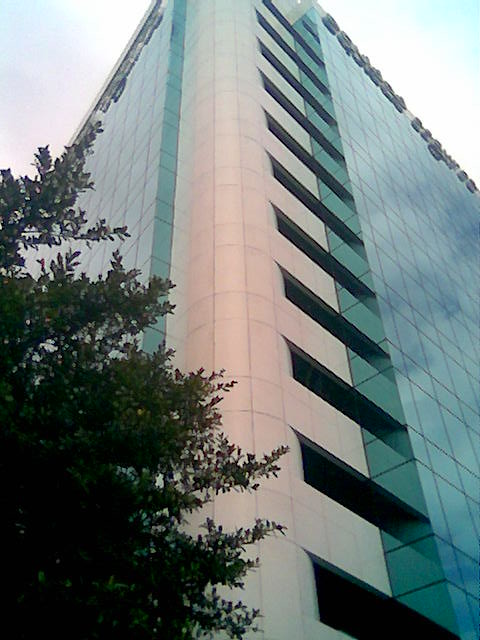The photograph showcases a very modern, multi-story building with a glass facade from a low-angle perspective, emphasizing its towering height against an overcast sky. The building, which appears to be at least 15 stories tall, features hundreds of square windows that reflect a blue hue, suggesting a seamless geometric pattern. The structure has a rounded concrete corner on the left, adding to its contemporary aesthetic. Dominating the lower left side of the image is a large, leafy green tree that partially obscures the building's windows. This natural element contrasts with the sleek, urban design of the building. The top of the building bears some unreadable writing, likely the name of the company that owns it. The sky behind is a mix of white and blue, contributing to the overall modern yet slightly dreary atmosphere of the scene.